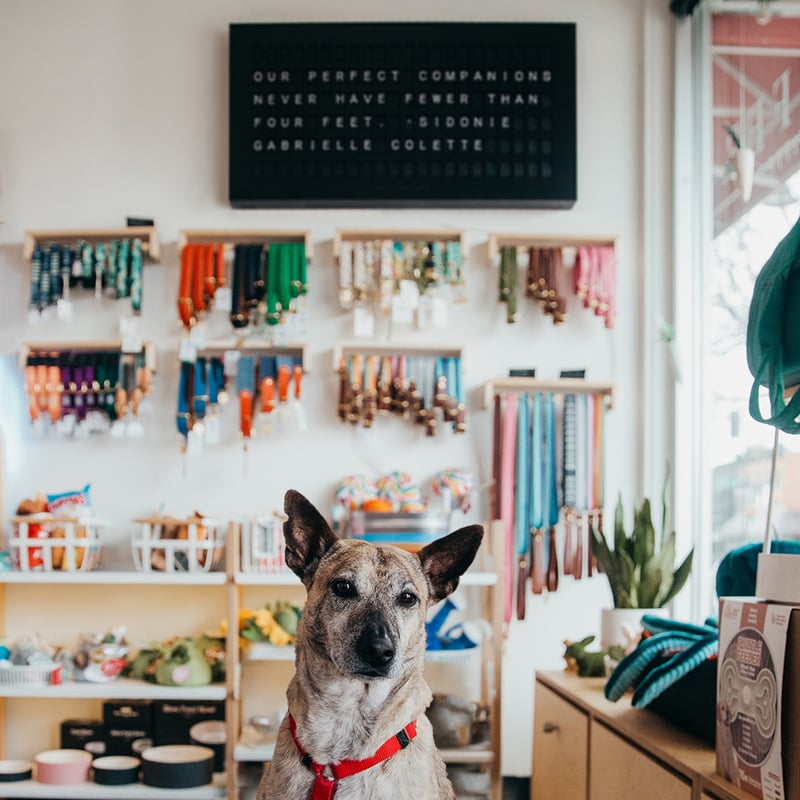In this photograph taken inside a pet store, the central focus is a light-colored dog resembling a German shepherd, with pointed ears, black nose, and eyes, situated at the bottom center of the image. The dog is wearing a red collar and sits in the foreground, facing the camera but gazing into the distance. Behind him, a white wall is adorned with a variety of collars and leashes of different lengths and colors. Shelves housing dog bowls, pet toys, and food items are visible, with some depth of field blurring these background details.

On the right side of the image, a table carries a small snake plant and some blue bags. A counter with a plate glass window runs along the right edge, allowing sunlight to stream into the store. Above the leashes, a black sign with white inset letters reads, "Our perfect companions never have fewer than four feet. — Sidonie Gabrielle Colette." This sign stands out prominently within the store's decor.